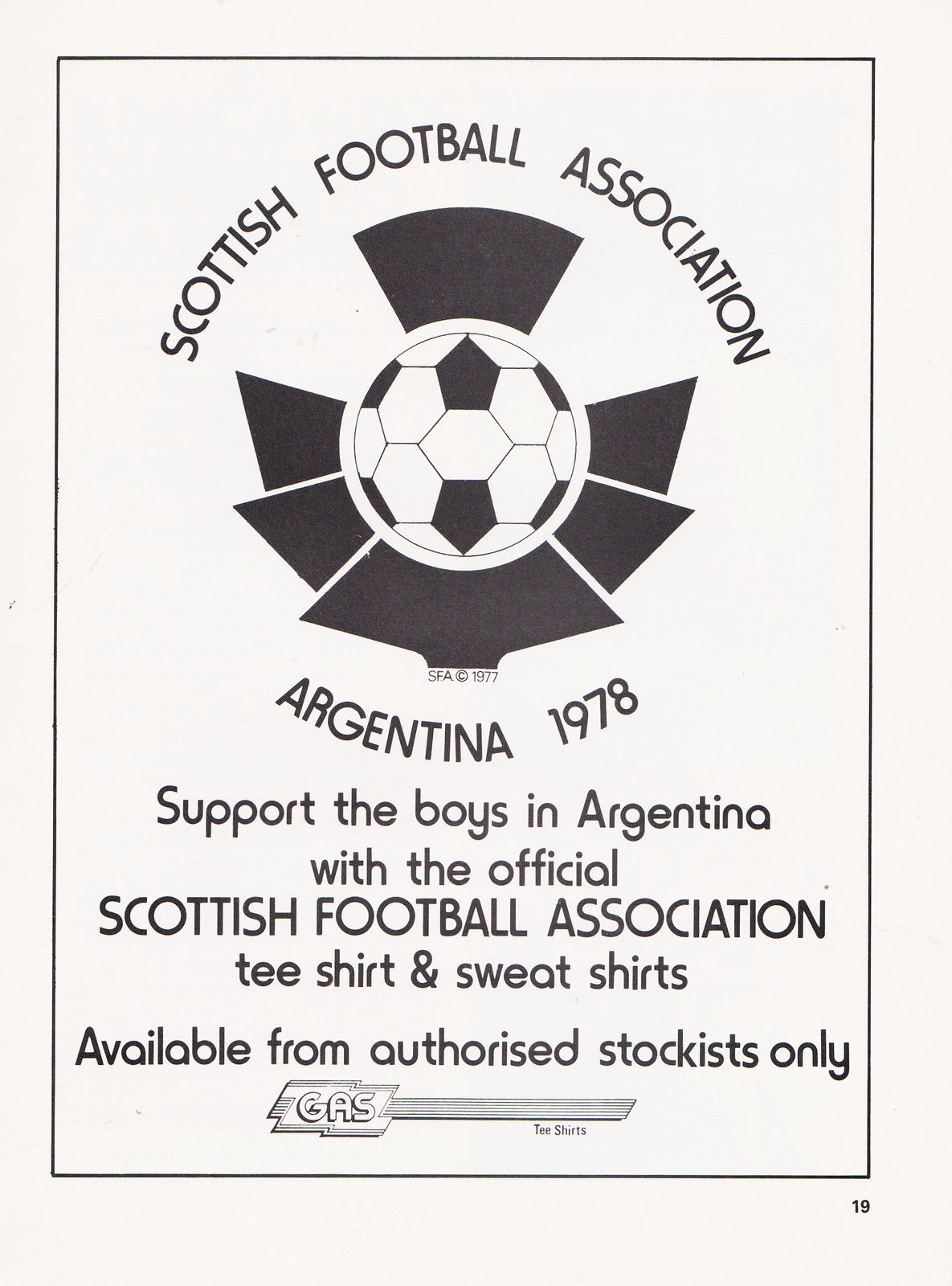This image is a highly detailed page from a football magazine, marked as page number 19 in the bottom right corner. The page features a predominantly white poster with black text and logos. At the top, the text "Scottish Football Association" is prominently displayed in a semicircle. Centered below this text is a black and white soccer ball with wing-like extensions radiating to the bottom right, left, and top, accompanied by the text "Argentina 1978" beneath it. Further down, the text encourages readers to "support the boys in Argentina with the official Scottish Football Association t-shirts and sweatshirts available from authorized stockists only." At the very bottom of the page, there's a logo featuring the text "gas," likely representing the brand responsible for the official merchandise. The entire poster is enclosed within a thin black border, adding to its structured presentation.